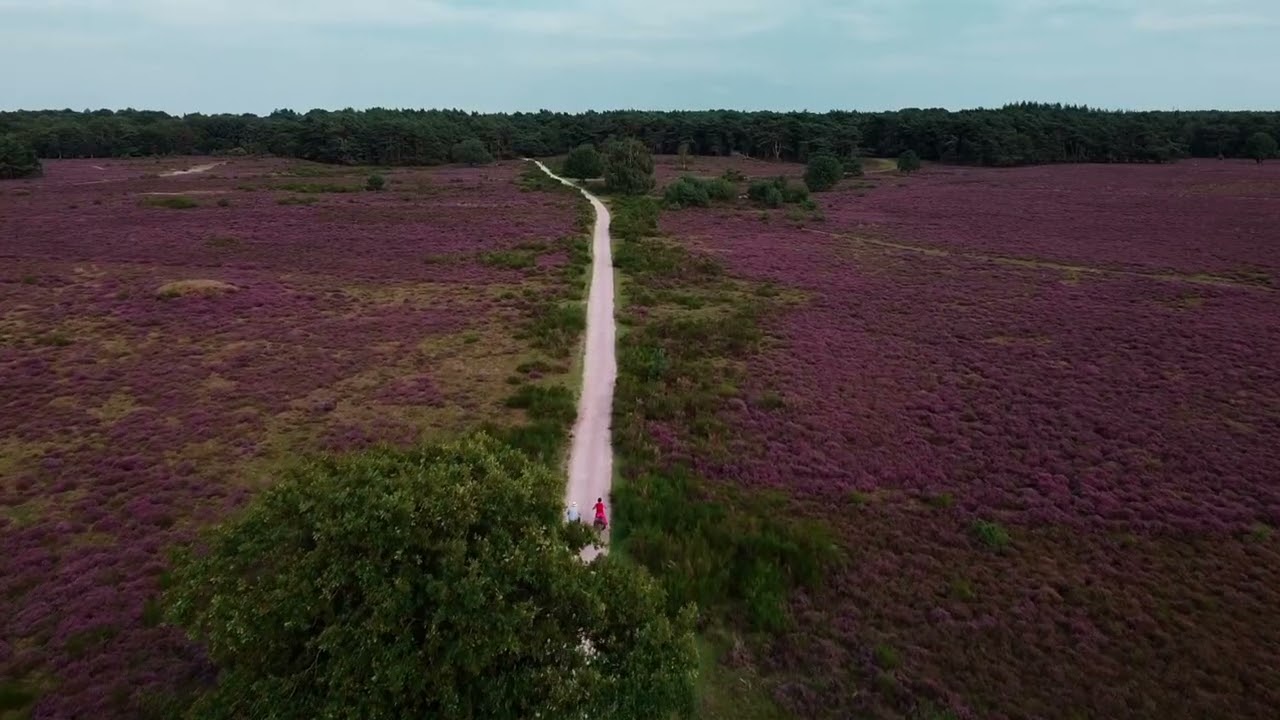This color photograph, captured from a low-flying drone, provides a detailed aerial view of a picturesque landscape. Dominating the scene is a sandy-colored, dirt road that cuts centrally through a diverse terrain, extending straight ahead until it disappears into a dense forest that spans horizontally across the top of the image. The road is slightly obscured by large shrubberies and trees in the lower left center, enhancing the natural feel of the image.

In the foreground, to the left and right of the road, the ground is covered with a purple grass-like vegetation interspersed with green shrubs, adding a striking contrast to the earthy tones of the road. Further left and right, the area is bordered by brown topsoil or gravel. The clear blue sky in the background, indicative of the middle of the day with no cloud cover, frames the lush green forest that stretches across the horizon.

On the road, two figures can be seen; one appears to be a woman in a red top, while the other is dressed in white, possibly wearing a white hat. Though it's ambiguous whether they are riding motorcycles, bikes, horses, or simply walking due to the height from which the photo is taken, their presence adds a dynamic element to the otherwise serene landscape. There are no other objects or text in the image, allowing the viewer to fully appreciate the natural beauty of the scene.